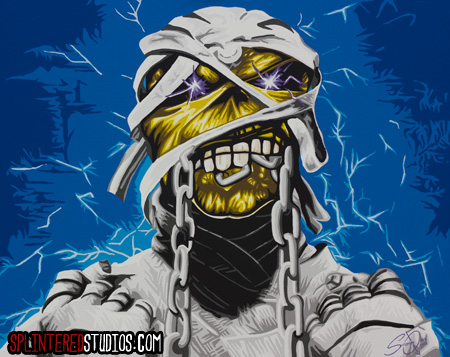The image is a highly detailed cartoon illustration, reminiscent of Iron Maiden album art, prominently featuring a mummy-like figure with an eerie, alien appearance. The creature's decayed yellow face peers through gaps in its white bandages, revealing large, glowing eyes that vividly shine with light, and a grimace with clenched white teeth biting down on a metal chain. The mummy’s hands, clad in gloves, are raised to shoulder height, as if poised to break free. Surrounding the figure is a dynamic background of blue hues, transitioning from light to dark, with white and light blue electrical sparks and lightning crackling prominently. A watermark reading "splinteredstudios.com" is positioned at the bottom right of the image, indicating the artwork's origin. The overall composition exudes a powerful, electrifying energy, combining elements of horror and heavy metal aesthetics.